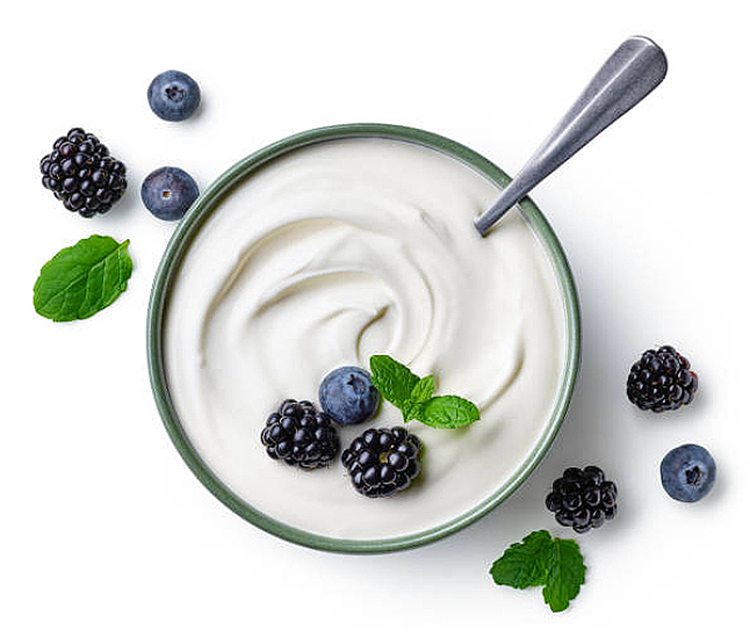This overhead, close-up image captures a large green bowl filled with plain, white yogurt, exhibiting a swirling pattern. A silver spoon is placed in the upper right-hand corner of the bowl. Within the yogurt, located near the bottom, are two blackberries, one blueberry, and a green mint leaf. The berries appear ripe and add a pop of color to the creamy yogurt. Surrounding the bowl, there is a symmetrical arrangement: to the upper left, there is one green leaf, two blueberries, and one blackberry; to the bottom right, there are two blackberries, a blueberry, and another mint leaf. The entire scene is set on a bright white background, with the bowl casting subtle shadows that emphasize the brightness of the yogurt and the vibrancy of the fruit.